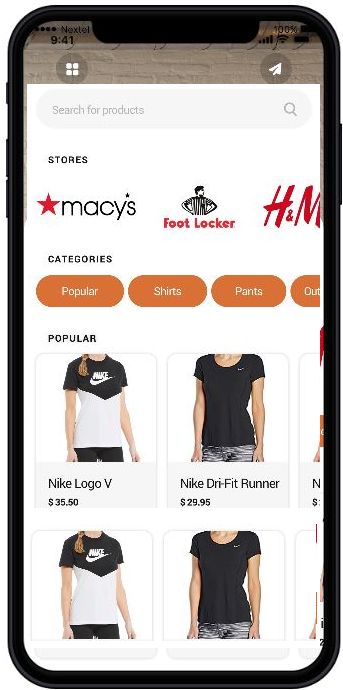This screenshot captures a storefront webpage featuring a clean and organized layout. At the top of the page, there is a light gray search bar prompting users to "Search for products," with a search button positioned on the right side. The main content area of the webpage is predominantly white.

Directly below the search bar, on the left side, the page displays a section labeled "Stores," showcasing three logos. Among these logos, Foot Locker and H&M are clearly visible. 

Further down, the page highlights "Categories," presenting four pill-shaped orange buttons with white text. The visible buttons include "Popular," "Shirts," and "Pants," with the fourth button partially cut off in the screenshot.

Beneath the categories, the "Popular" section features a grid layout displaying various product listings. The visible items in the first two rows include:
- A Nike product priced at $35.50.
- A Nike Dri-FIT runner priced at $29.95.

Only four products are visible in the grid due to framing, offering a snapshot of the available merchandise.